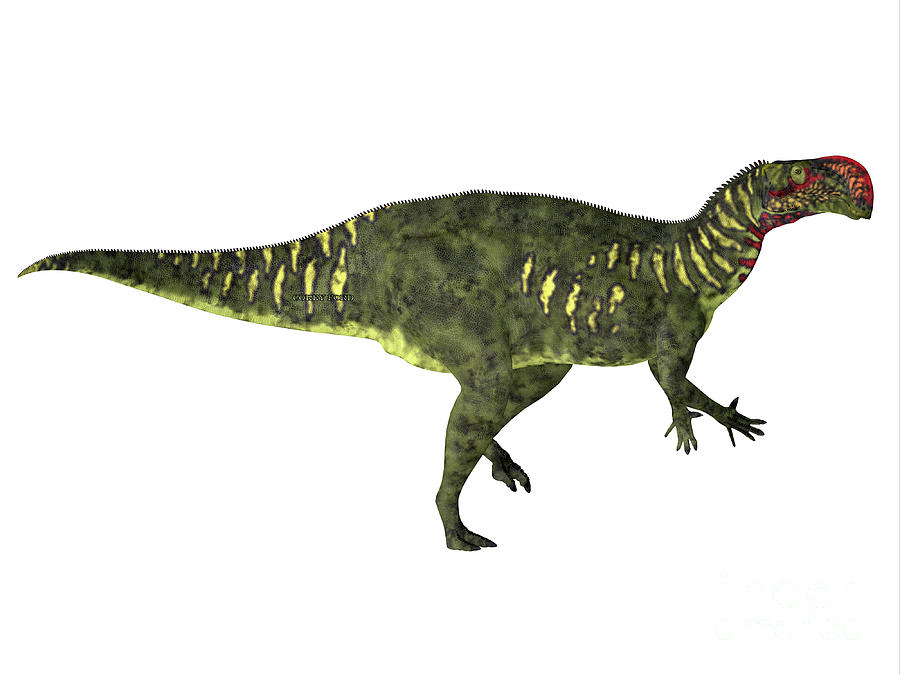This striking computer-generated image features a detailed, large green dinosaur standing on its two hind legs against a predominantly white background. The dinosaur is richly colored in varying shades of dark green, with darker green splotches and lighter green or lime green patches around what appear to be ear-like structures. It has an imposing figure with a slender tail that ends in a point and has a row of spiky hair running from the top of its head all the way down its back to the tail tip. 

The creature sports a unique, toucan-like beak with a curved, bird-like peak, which displays hues of red and orange. The red coloration extends to patches beneath the eyes and across the throat area, accentuating the animal's vibrant appearance. It has five-fingered hands held out in front, short arms, and eyes described as wide and prominently outlined in green and black. The body is adorned with yellow stripes along the sides and neck, giving the dinosaur a colorful, dynamic look. 

The overall likeness could be reminiscent of a miniaturized Tyrannosaurus Rex, with notably more slender legs and a more elongated, less massive head. While there appears to be a name in the image, it is unreadable but might read something like "Jeffrey Ford." Despite not being regarded as an exceptional image in quality, the details offer a vivid depiction of this imaginative prehistoric creature.